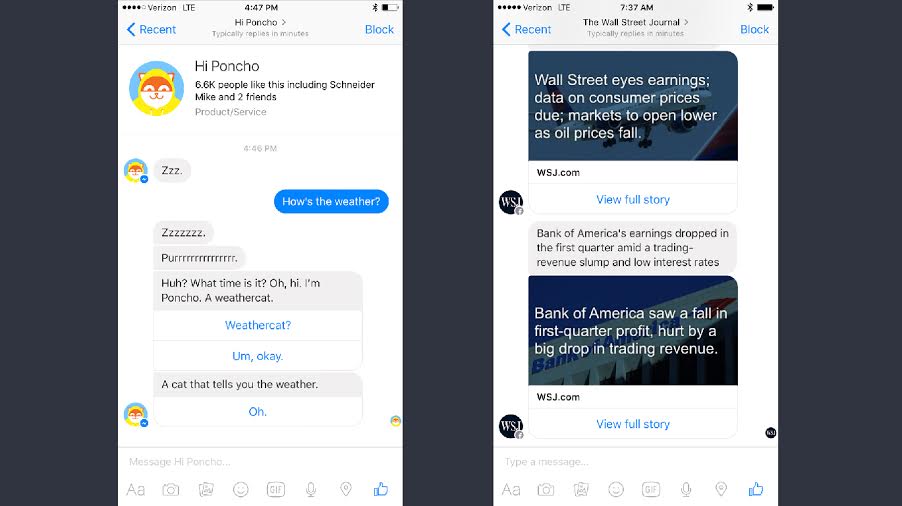Here is a cleaned-up and detailed descriptive caption for the images:

---

**Image Caption: Dual Screenshot of Mobile Interface Interactions**

The provided image is a side-by-side comparison of two screenshots from a mobile device, though the images have been poorly cropped and do not utilize the full screen space. Both images display an interface for interacting with AI chatbots, featuring various icons for typing messages, formatting text, taking pictures, inserting images, emojis, GIFs, using the microphone, sharing location, and liking comments.

**Left Screenshot: Weather Cat Poncho Interaction**
- The device shows a Verizon LTE connection with four out of five bars of cellular service. It is 4:47 p.m., Bluetooth is enabled, and the battery indicator is less than halfway charged.
- The chat screen is labeled "Recent" with an arrow pointing left and provides an option to block the contact.
- The conversation is with "Hi Poncho," an AI chatbot that typically replies in minutes. Poncho is depicted as a cat wearing a raincoat with its ears poking out. It has received 6.6 likes, including users Schneider Mike and two others.
- The service is described as a product service. In the chat, Poncho responds "zzzz" at 4:46 p.m. The user asks, "How's the weather?", to which Poncho replies sleepily with "Purr. Huh? What time is it? Oh, hi, I'm Poncho, a weather cat." The user is prompted to respond with "weather cat" or "okay."
- Poncho then describes itself as "a cat that tells you the weather." 

**Right Screenshot: Wall Street Journal Interaction**
- This screen similarly has recent chats and a block option, but it interacts with the Wall Street Journal bot.
- The chatbot, typically responsive within minutes, shares a news headline: "Wall Street eyes earnings data on consumer prices due markets to open as oil prices fall." Users can click a link to view the full story.
- Another news bulletin follows: "Bank of America's earnings dropped in the first quarter amid a trading revenue slump and low interest rates. Bank of America saw a fall in first-quarter profit hurt by a big drop in trading revenue." Again, there is an option to view the full stories.

Both screenshots suggest interaction with bots within an application, capable of providing specialized information ranging from weather updates to financial news.

---

This format enhances the original description by providing a structured and detailed narrative of the images, clarifying the context and functionality depicted.